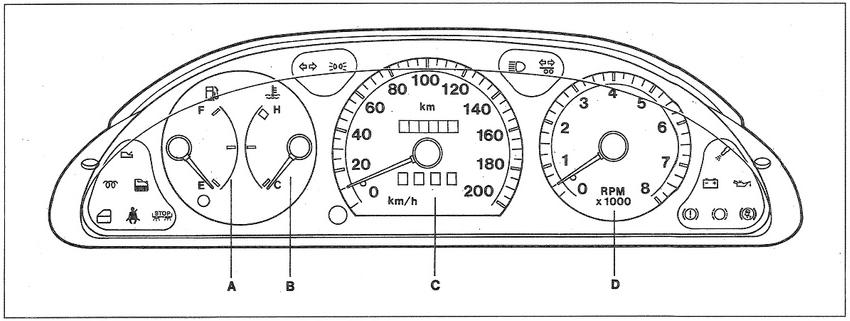This black and white illustration offers a vintage-style, detailed view of a car's dashboard, reminiscent of those found in an owner's manual. The image, likely from several years ago, meticulously labels various dashboard components, such as the speedometer, tachometer, fuel gauge, and temperature gauge. It also highlights the different warning lights that a driver might encounter, including indicators for high beams and other essential notifications. The labels A, B, C, and D suggest that the illustration corresponds with further explanations within the manual. Rectangular in shape, the image measures approximately five inches across and two inches vertically, capturing a comprehensive but concise representation of the dashboard for easy reference.